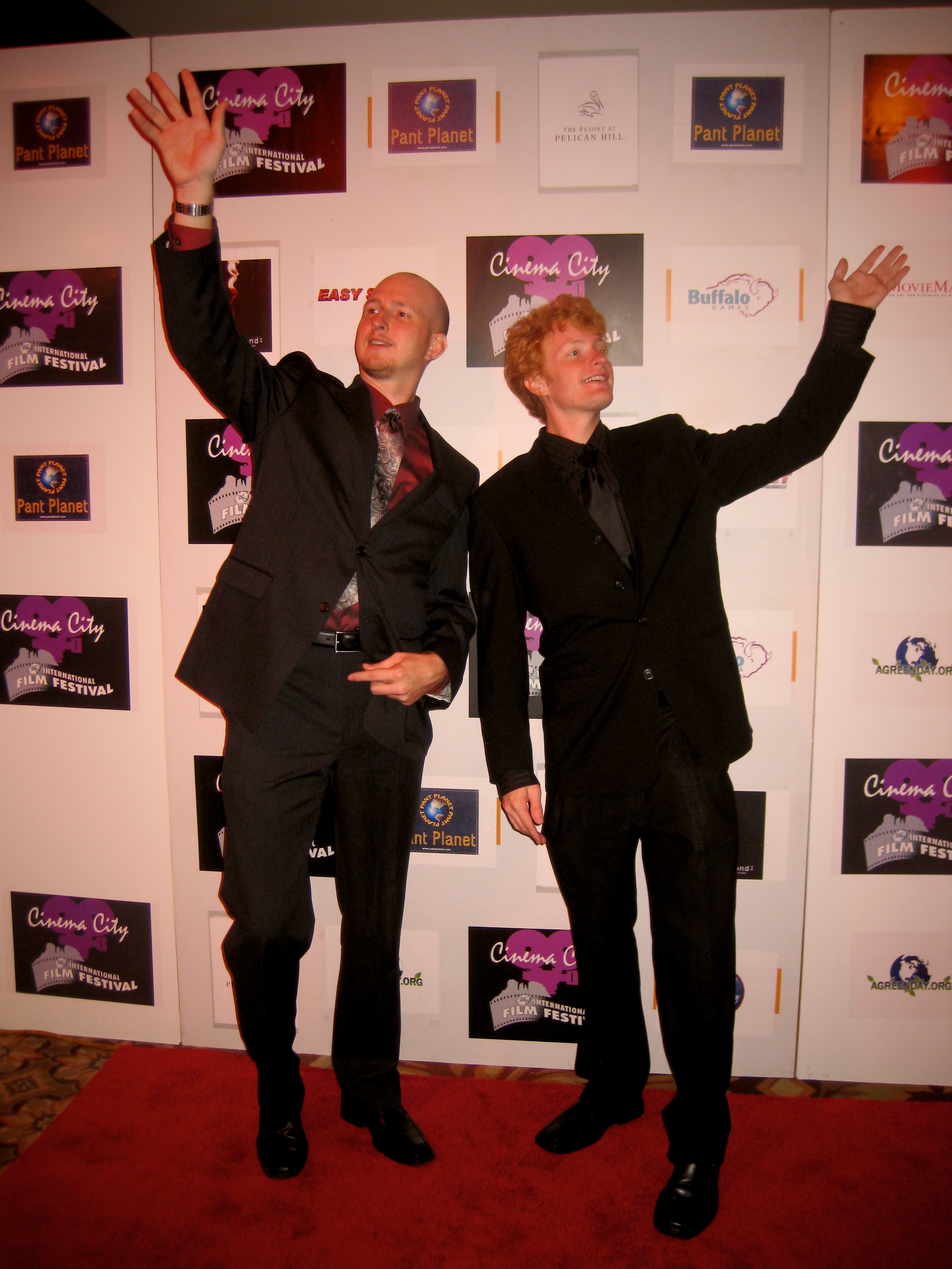This image portrays two young men standing on a red carpet at what is clearly the Cinema City International Film Festival, as evidenced by the repeated festival posters on the press backdrop behind them. Both men are impeccably dressed in suits; the man on the left sports a gray suit with a burgundy shirt and silver tie, along with a watch on his right wrist and a balding head, while the man on the right dons a black suit with a black shirt and gray tie, with orange hair. They are both waving— the left man with his right hand and the right man with his left hand— creating a mirrored pose. The red carpet overlays a brown carpet with a diamond-like design, and smaller advertisements for "Plant Planet," "Easy Something," and "Pelican Bill" complement the Cinema City posters. The scene suggests that these individuals are likely actors or directors associated with the film festival, engaging with onlookers or paparazzi.